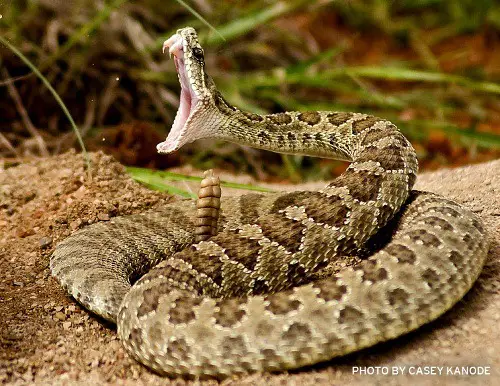This nature photograph, credited to Casey Kanode, vividly captures an agitated rattlesnake in its natural outdoor habitat, likely within a wooded area during daylight. Prominently featuring the large snake, the close-up shot reveals its wide-open mouth, displaying curved, pinkish fangs. The rattlesnake is posed in a coiled position with its rattler standing erect, clearly visible just below its head. Its eyes are nearly entirely black and positioned towards the back of its head. The snake's tan body is adorned with a distinguishing pattern of light brown and darker brown diamond-shaped markings, which transition to a stripe-like design closer to its tail. The texture of the snake's oval scales further enhances the detail captured in the photograph. The background features a fine, brown soil surface with stalks of green plants emerging, adding to the naturalistic setting. Additionally, a thin stalk of grass is positioned near the front of the rattlesnake's mouth. This photograph, possibly intended for a textbook or website, offers a striking and detailed portrayal of the rattlesnake in its environment.